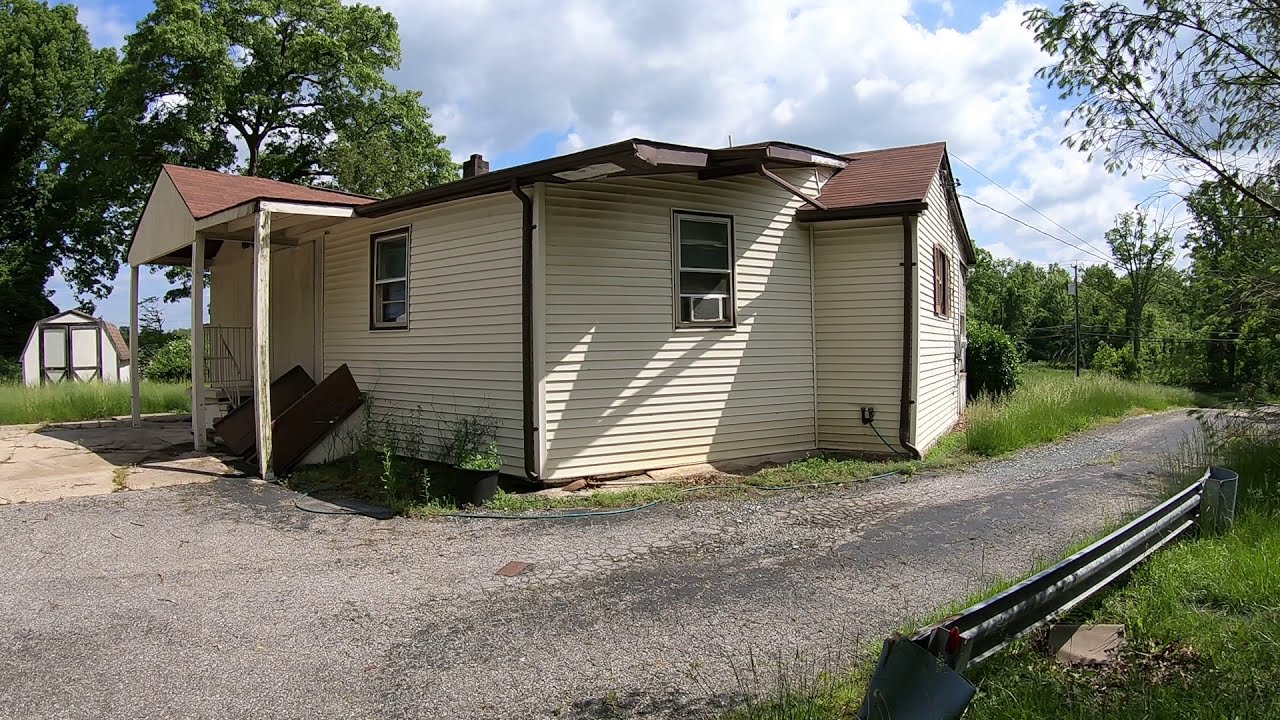This photograph captures a small, somewhat rundown beige house situated by a narrow, old street. The house has small square windows visible on at least two sides and a short, brown roof. You're looking at the corner of the house where two sides meet; one extends to the left and the other to the right. The front porch features a large, ambiguous brown object leaning against it. A hose runs along the exterior of the house, and an air conditioning unit is installed in one of the windows. 

In the background to the left, there's a beige and brown shed. Surrounding the house is an expanse of tall, untamed grass, and numerous trees frame the scene from behind. The overcast sky above is filled with a mixture of puffy white and gray clouds, with patches of blue peeking through. A tree's branches intrude into the upper right corner of the image, while a piece of metal is partially embedded in the ground at the lower right. Overall, the picture portrays a quaint, solitary house amidst a slightly overgrown and naturally lush setting.